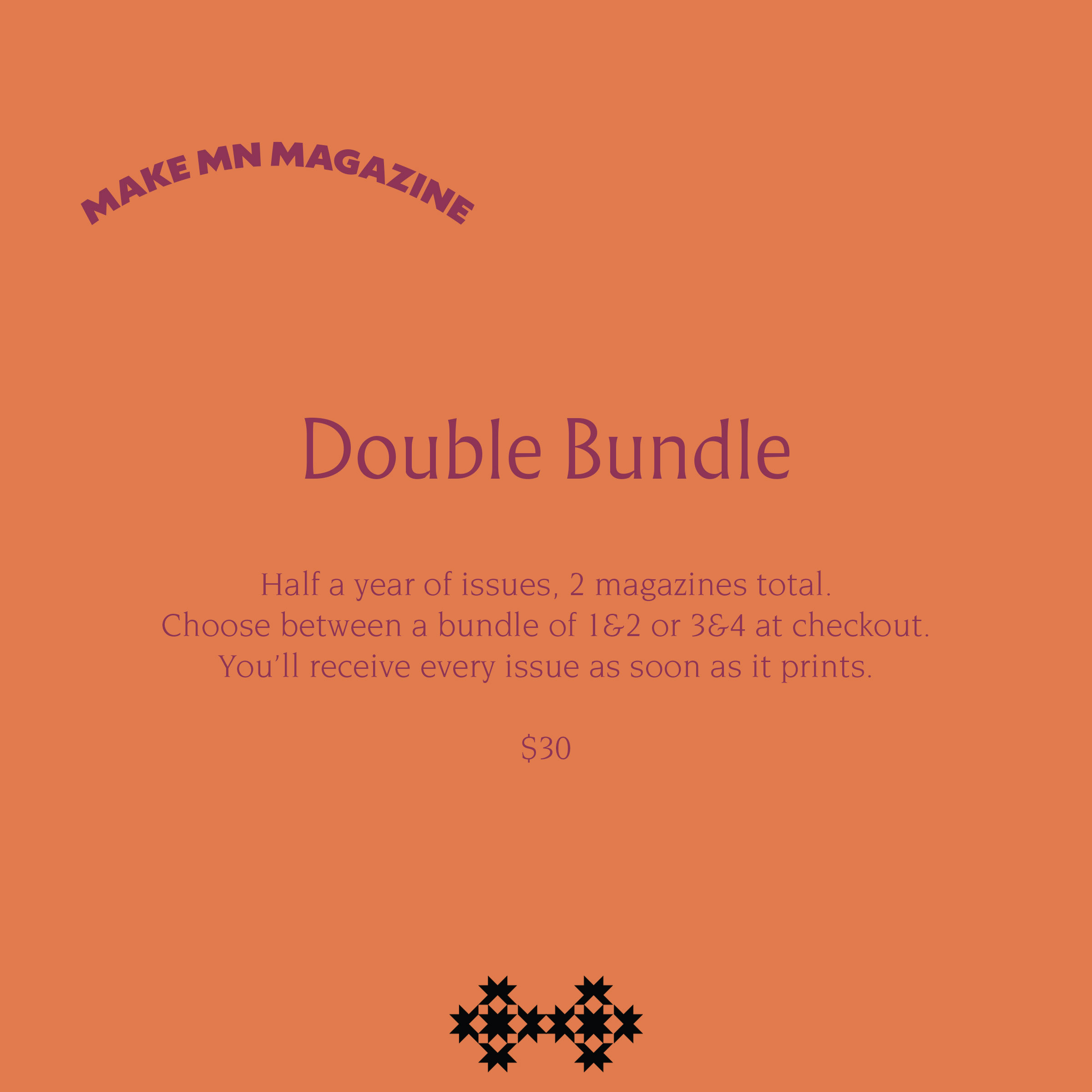The advertisement features a vibrant orange background with text arranged in a visually appealing layout. At the top, an arch-shaped text in purple, all uppercase, reads "MAKE MN MAGAZINE." Centered in the middle of the page, bold and in purple, is the headline "Double Bundle" with capital D and B. 

Beneath this, additional text in a typewriter-style font provides details about the offer: "Half a year of issues, two magazines total. Choose between a bundle of one and two, or three and four at checkout. You'll receive every issue as soon as it prints." Following a few blank spaces, the price "$30" is listed. At the bottom of the page, there is a distinctive design composed of two interconnected stars, adding a unique touch to the advertisement.